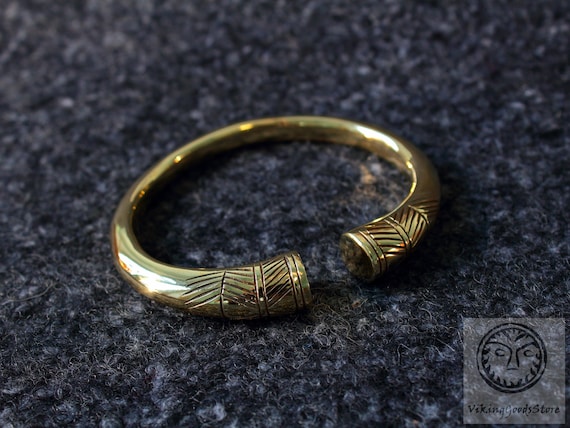The image is a close-up photo of a gold-colored, open-ended brass ring or bangle, characterized by its circular shape that does not close completely. The unfinished ends of the circle feature intricate engravings or etchings that resemble leaves or other delicate designs. The focus is sharp at the front of the ring, showcasing the details of the engravings, while the back portion fades into a gentle blur, adding depth to the visual. The object is laid atop a dark gray, textured cloth with light gray speckles, reminiscent of felt. In the bottom right-hand corner of the image, a translucent logo is visible, featuring a circle with a face, and beneath it the words "Viking Goods Store." This setup, potentially captured in a light box with studio lighting, suggests that the image could be an advertisement for a jewelry company, showcasing what appears to be a bracelet.